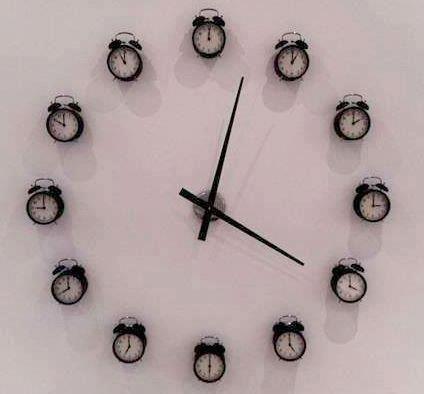This image features an innovative and intriguing wall clock, potentially a homemade creation, displayed on a pristine white background. The clock is an arrangement of 12 individual small, black analog alarm clocks. Each alarm clock represents a numeral on a traditional clock face, positioned at the corresponding hour placements. For instance, one clock marks the 12 o'clock position, one at 3 o'clock, another at 6 o'clock, continuing in a circular formation encompassing the full dozen.

Each alarm clock sports a classic design, complete with twin bells mounted on top. Their faces are stark white, creating a striking contrast with the black hour and minute hands, and the black hour markings. Notably, there are no numerical indicators on the faces of these alarm clocks. The setup as a whole is meticulous, with each clock synchronized to display the same time—approximately 4:03. This artistic and unconventional arrangement brings a unique and visually captivating twist to the concept of a wall clock.